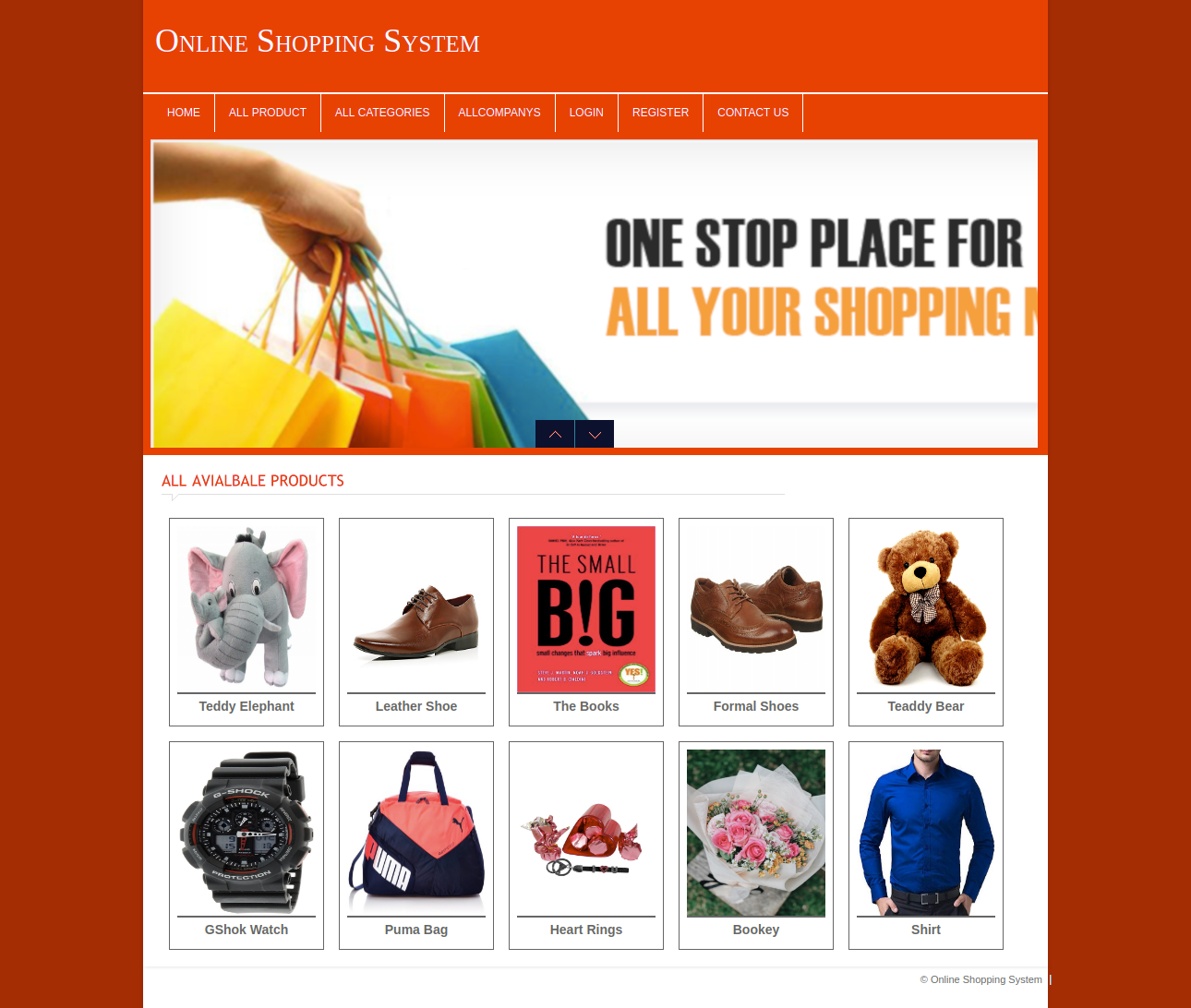**Detailed Caption for the Image:**

The image captures a website interface for an Online Shopping System. The layout features darker red borders on both the left and right sides. At the top center of the page, an orange-tinged header displays the text "ONLINE SHOPPING SYSTEM" in bold white capital letters. Beneath this header, a thin horizontal line extends across the page, from one red border to the other.

Directly below this line, a navigation menu is displayed, listing the following options from left to right: "Home," "All Products," "All Categories," "All Companies," "Login," "Register," and "Contact Us."

A prominent white banner occupies the area below the navigation menu. This banner features an image of a person's right arm extended outward, holding a variety of shopping bags in different colors—yellow, red, orange, green, and blue. Accompanying this visual are the words "One Stop, Place For" in black text, followed by "All Your Shopping" in orange-yellow text, which appears to be cut off at the end.

The main content section of the page has a white background with a headline that reads "All Available Products." Notably, the word "Available" is misspelled as "AVIABALE." 

This section is organized into two rows of product listings, each containing five squares that showcase different items. 

- **Top Row:**
  1. Teddy Elephant
  2. Leather Shoe
  3. Books
  4. Formal Shoes
  5. Teddy Bear

- **Bottom Row:**
  1. G-Shock Watch (misspelled as "G-SHOK Watch")
  2. Puma Bag
  3. Heart Rings
  4. Bookie
  5. Shirt

Overall, the image provides a thorough representation of the website's design, showcasing its color scheme, navigation options, and a sample of available products.